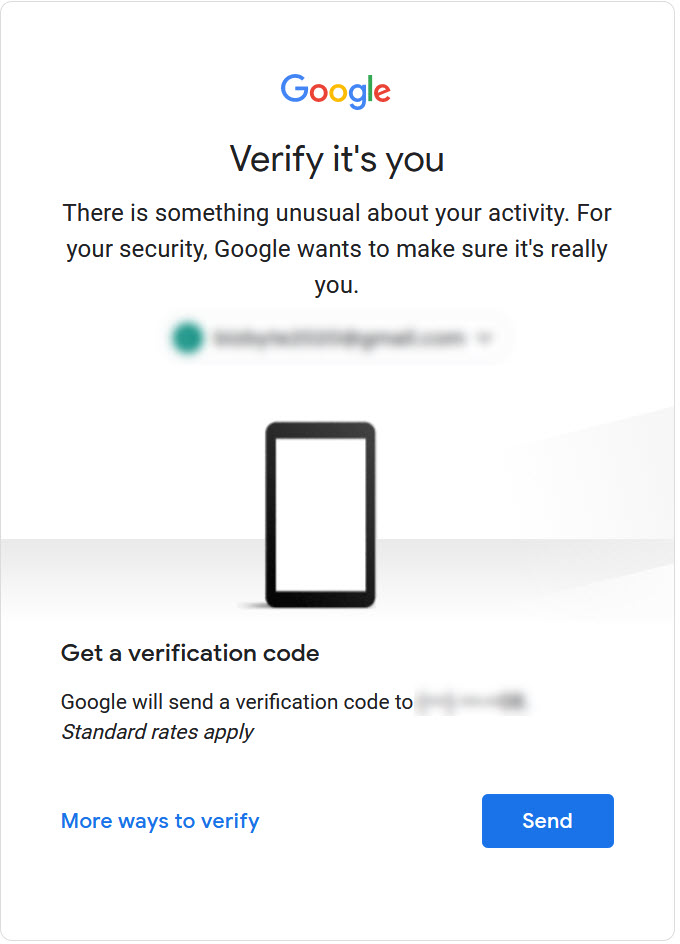The image depicts a Google verification page designed for phone verification, emphasizing the importance of securing user accounts. At the top of the page, the iconic Google logo in its blue, red, yellow, and green colors is prominently displayed. Below the logo, a bold and clear message reads "Verify it's you," followed by a cautionary notice stating, "There's something unusual about your activity. For your security, Google wants to make sure it's really you."

The user's email address is shown but is completely blurred out for privacy. Centered on the page is an image of a smartphone with a black edge and a white screen. Beneath the phone image, the instructions "Get a verification code" are displayed. Google indicates that a verification code will be sent to the user's phone, though the phone number is blotted out for security reasons. It is also noted that standard messaging rates apply.

At the lower left of the page, there is a clickable link labeled, "More ways to verify" in blue text. On the bottom right, a blue box with the text "Send" in white lettering is present, inviting the user to proceed with receiving their verification code.

Overall, the scene highlights the process of securing a Google account through phone verification. In the background narration, there is a mention of a dog barking, indicating that people have arrived home.